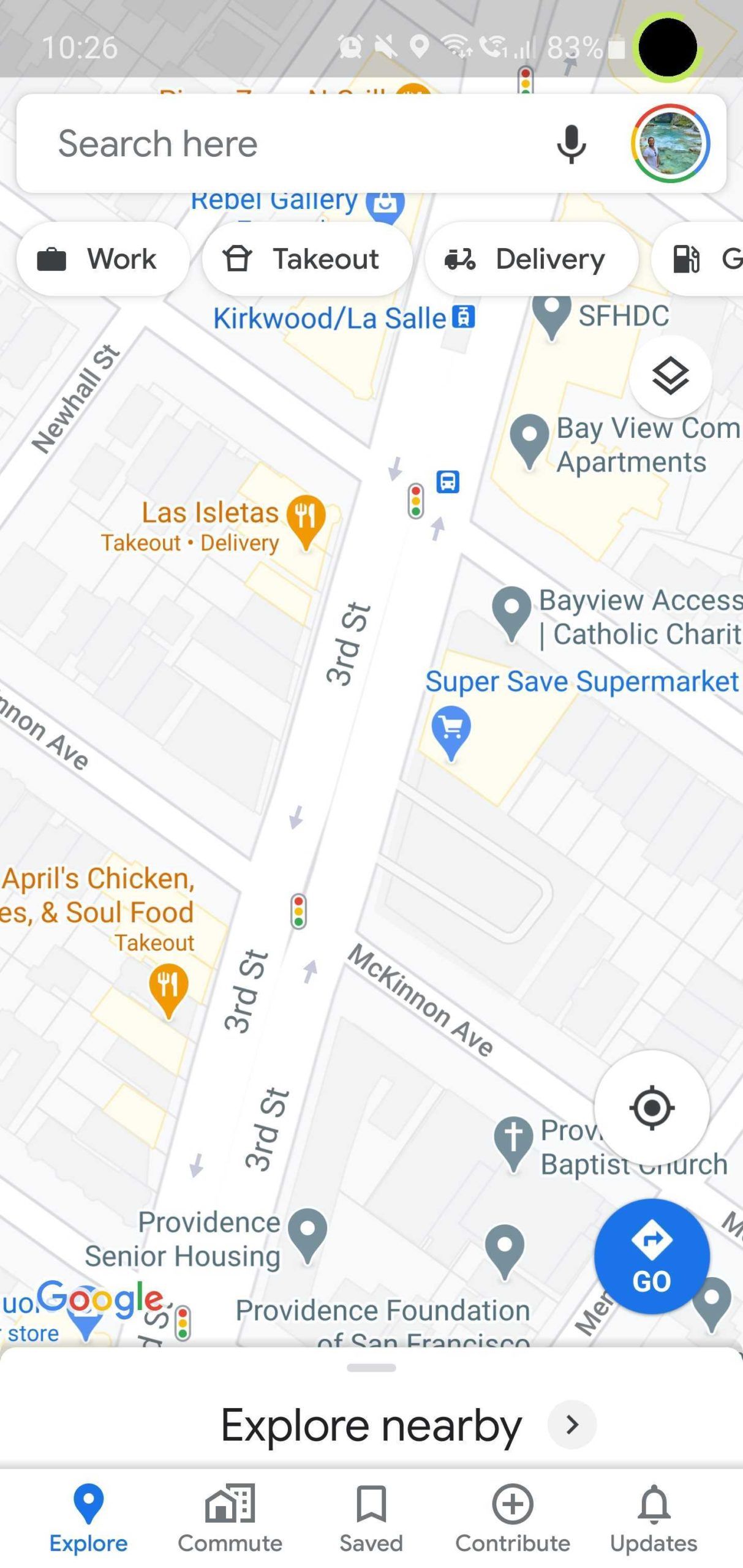This image depicts a Google Maps interface displayed on an iPhone screen, showcasing various features and indicators. The iPhone's battery life is prominently shown at 83%, with the current time marked as 10:26. At the top of the screen, a white search bar invites users to 'search here' and includes an image of a microphone for voice searches. Adjacent to the search bar is a profile picture characterized by green and blue hues.

Central to the image is a detailed and close-up view of a map. The map includes markers for 'Work,' 'Takeout,' 'Delivery,' and 'Gas,' though only the letter "G" of 'Gas' is visible alongside a gas tank icon. A prominent main road runs diagonally through the middle of the map. Notable locations highlighted on the map include a "Super Save Market" and a soul food takeout establishment.

The interface clearly indicates the use of Google Maps through the Google logo on the bottom left, represented in its distinct blue, red, gold, blue, green, and red colors. Below the map, a section labelled "Explore nearby" with a right-pointing arrow appears, followed by another "Explore" section.

Additional navigation options such as "Commute," "Saved," "Contribute," and "Updates" are visible beneath these sections, indicated by respective icons. A blue pin is featured prominently on the map. At the map's periphery, a blue circle contains a white diamond shape with an arrow in its center. Lastly, a distinct lime green circle with a black center stands out at the top of the display.